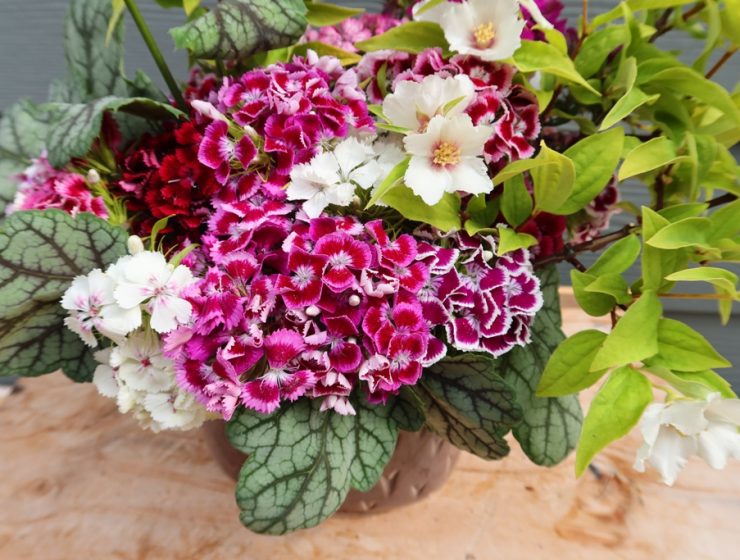This close-up photograph captures a stunning and detailed flower arrangement, almost resembling a bouquet, placed on a wooden tabletop. The flowers are diverse in color, predominantly showcasing a harmonious mix of white, red, and purplish-pink hues. The arrangement features a variety of blooms, including white flowers with yellow centers scattered throughout, and red flowers, possibly carnations, prominently mixed in the middle. Purple and pinkish tones blend seamlessly with the white and red flowers, creating a vivid and visually pleasing composition. Green leaves frame the arrangement, with larger, vine-like leaves at the base and smaller, lighter green leaves towards the top right. The flowers are complemented by a clay pot, which adds an earthy aesthetic to the overall display. The wooden tabletop beneath the arrangement, though slightly out of focus, enhances the natural and rustic charm of the setting.